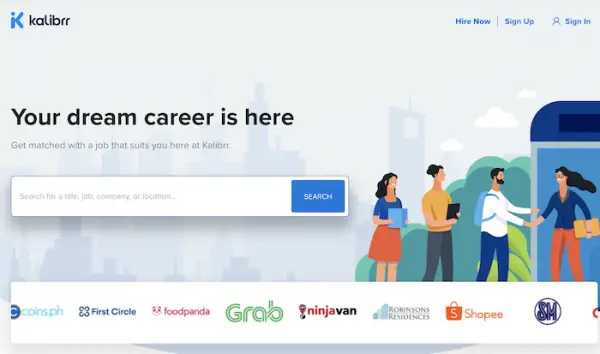Screenshot of a web page from Kalibrr, featuring a combined 'I' and 'K' logo in blue at the top left. To the right is the name "KALIBRR" in black letters. Further to the right, navigation options include "Hire Now," "Sign Up," and "Sign In" in dark blue. The center-left of the screen displays the tagline, "Your dream career is here. Get matched with a job that suits you here at KALIBRR." Below this tagline is a large white search bar with a blue search button.

On the right side, animated illustrations of people are featured: 
- A woman with a blue shirt, red skirt, and dark hair holding a folder.
- A tall man in a yellow shirt and gray pants with dark hair also holding a folder.
- A man with dark hair and a beard, wearing a white shirt, blue backpack, and blue pants, shaking hands with a woman with long dark hair, glasses, a blue shirt, and red pants, who is holding a folder as well. Behind these figures is a blue building with green trees.

At the bottom of the screen is a white bar displaying various brand names: "Coins.ph," "First Circle," "Foodpanda," "Grab," "Ninja Van," "Robinsons Residences," "Shopee," and "SM."